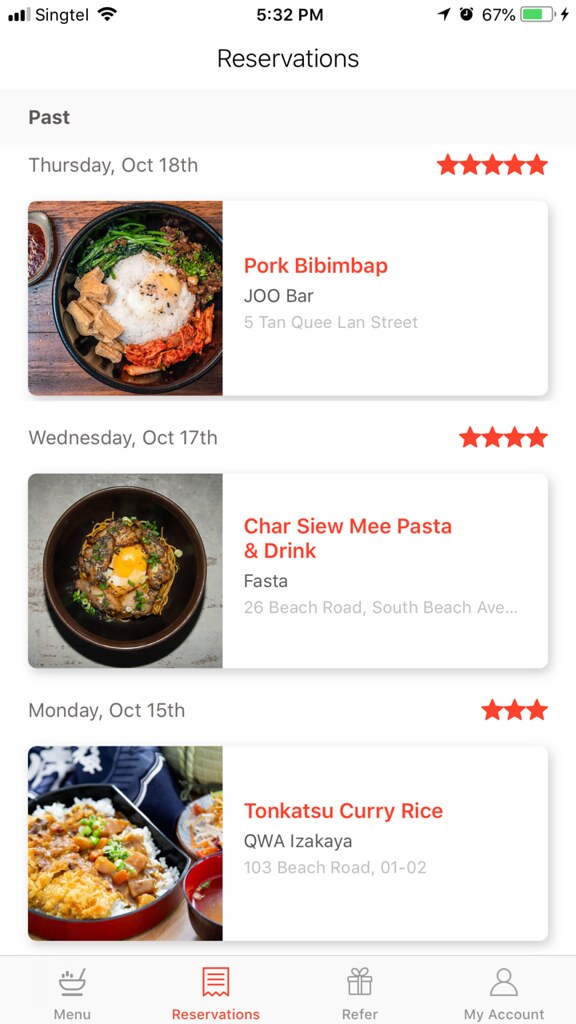A detailed screenshot of a mobile phone display highlighting the "Reservations" section of a food-related application. The status bar at the top indicates the phone's relevant details: the connection is through Singtel, with signal strength at three bars, the time displayed as 5:32 p.m., and the battery at 67% charge.

Immediately below the status bar, the screen shows the title "Reservations" with a gray underline and a "passed" label within it. The main content comprises three reservation cards showcasing different dining experiences:

1. **Top Card:**
   - **Date:** Thursday, October 18th
   - **Rating:** 5 red stars on the right
   - **Dish:** A visually appetizing black dish of bibimbap featuring a fried egg at the center, complemented by green vegetables, an element with red sauce, and noodles on the left.
   - **Details:** Pork Bibimbap from "Jew Bar" located at 510 Q Lawn Street

2. **Middle Card:**
   - **Date:** Wednesday, October 17th
   - **Rating:** 4 stars
   - **Dish:** A rustic shallow brown pottery bowl containing a pasta dish with brown sauce and a fried egg in the center.
   - **Details:** Char Siu Mee Pasta and Drink from "Fosta" found at 26 Beach Road, South Beach Avenue

3. **Bottom Card:**
   - **Date:** Monday, October 15th
   - **Rating:** 3 red stars
   - **Dish:** An elegant red lacquered dish with a black interior holding white rice accompanied by curry with apparent chunks of chicken and tofu.
   - **Details:** Tonkatsu Curry Rice from "KWA Izakaya" located at 103 Beach Road, Q1, Q2

At the very bottom of the screen, a gray navigation bar presents four selectable options:
   - **Menu:** Represented by a bowl with a fork
   - **Reservations:** Highlighted in red with a red piece of paper icon
   - **Refer:** Depicted with a gift box tied with a bow
   - **My Account:** Indicated by an outline of a person

This detailed description captures all the vital visual and textual information present in the screenshot.